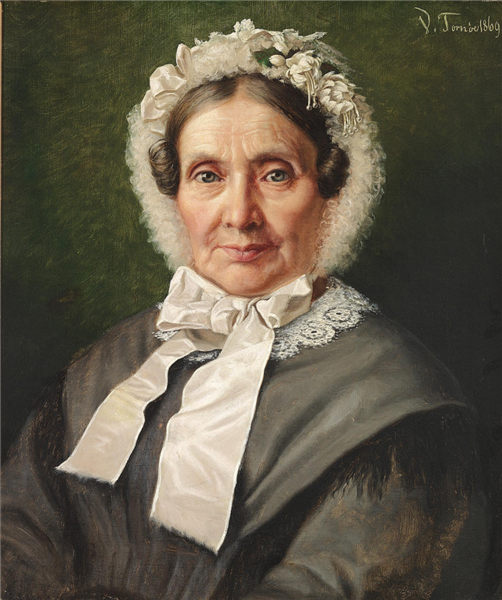The painting depicts an elderly Caucasian woman, likely around 67 years old, captured in an old-style painted portrait. Her deep wrinkles and stern expression lend gravitas to her visage. She has short, dark brown hair styled into small buns at the sides of her head, near her eye level, partially covered by a white bonnet. The bonnet is intricate, adorned with ribbons, flowers, lace, and fluffy material, tied under her chin with a large bow. Her eyes appear light grey to greenish, complementing her drab, old-fashioned attire.

She is dressed in a bulky, dark grey to black outfit, likely a dress, with prominent seams at the elbows and a white filigree lace mesh around her neck. The portrait captures her from the middle of her torso up, highlighting her elaborate bonnet and stern demeanor.

The background is a blend of green and dark hues, creating a gradient effect that makes the central figure stand out. There are scratchy yellow highlights against the green backdrop. In the top right-hand corner of the painting, there is a signature, partially legible as starting with "VT" followed by the year "1809," though the full details are difficult to make out. The overall composition suggests this is a meticulously crafted portrait from the early 19th century.